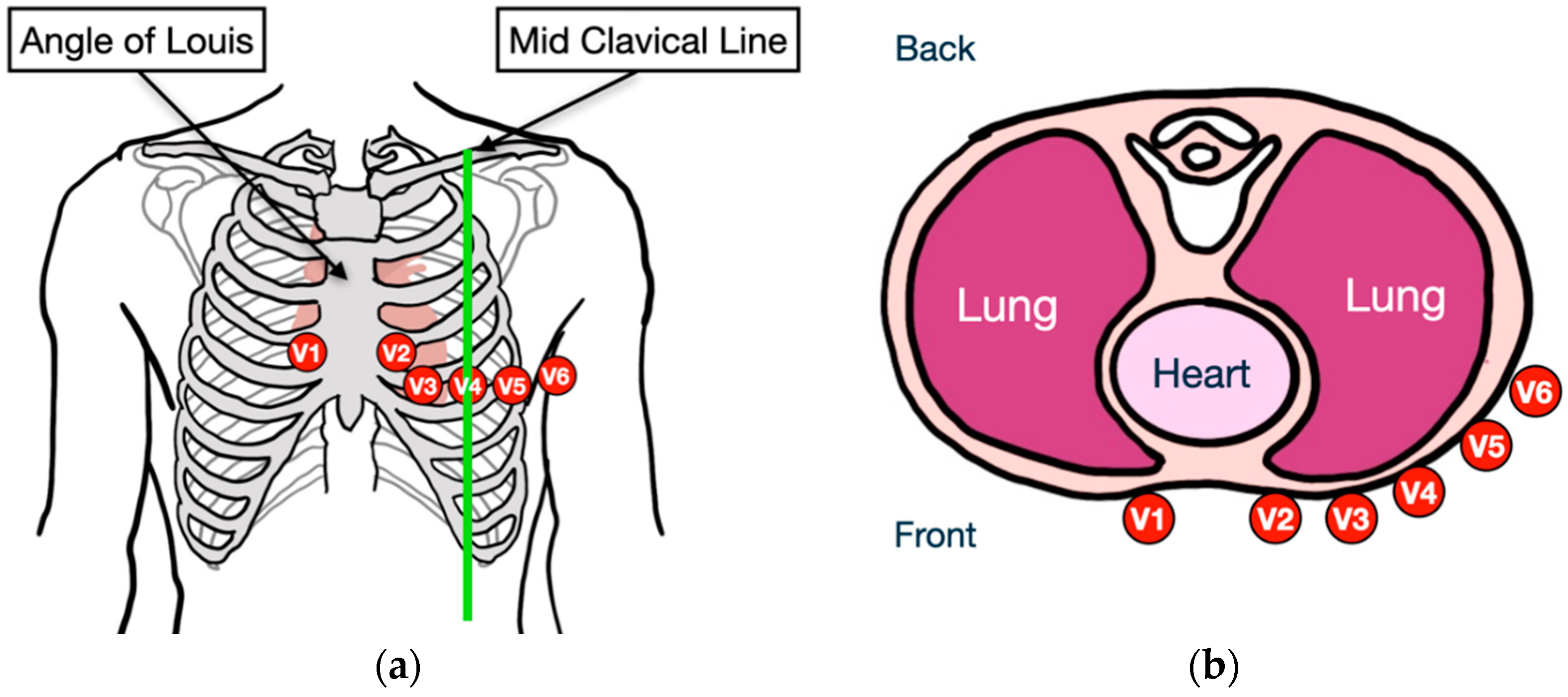This detailed medical drawing consists of two distinct sections. On the left side of the image, there is an anatomical illustration of a human chest. Here, the outlines of two arms extend from the shoulders to the elbows, along with the chest contour delineating just below the arms down to above the waist. The ribcage is prominently featured in gray, with various anatomical labels marked throughout by small red circles containing white numbers and letters. A prominent banner at the top left reads "Angle of Louis," pointing toward the mid-rib area where the ribs meet at the sternum. Another white banner on the right identifies the "Mid Clavicle Line," directing attention to the slender clavicle bone in the shoulder area. 

Adjacent to this, on the right side, is a detailed drawing of the lung and heart. This illustration provides a top-down view, enclosed within an oval outline shaded in light pink. Inside this oval, the lungs are depicted in a darker pink, while the heart is centrally positioned in a lighter pink oval, detailed with black writing. The bottom of both illustrations features orange circles with letters and numbers ranging from one to six, indicating different anatomical levels for reference.